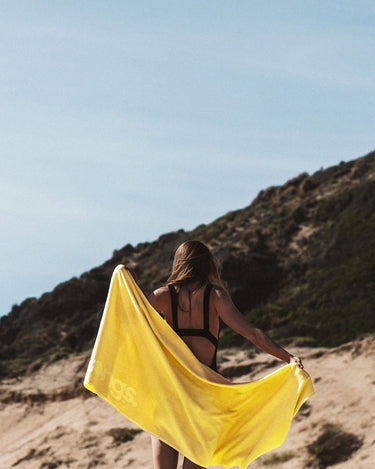In this vibrant, high-quality photograph, a young woman stands at the beach, facing away from the camera. Central to the image, her back is visible from her head down to her knees. She has long, brown hair, slightly tousled by the wind, and is wearing a black, open-back bathing suit. The woman is holding a bright yellow beach towel behind her, with its draped edges hinting at the moment she might wrap it around her shoulders. The towel features some unreadable font due to the way she holds it.

The background showcases a splendid natural scene: two-thirds of it is dominated by a clear blue sky. Below this sky lies a sloping hill, starting low on the left and rising higher to the right, covered with dense, dark green shrubbery. The hillside meets the sandy beach at the bottom of the frame, creating an inviting, beachy atmosphere. The photo adeptly captures the serene and scenic beauty of a day at the beach, emphasizing both the woman's presence and the picturesque surroundings.